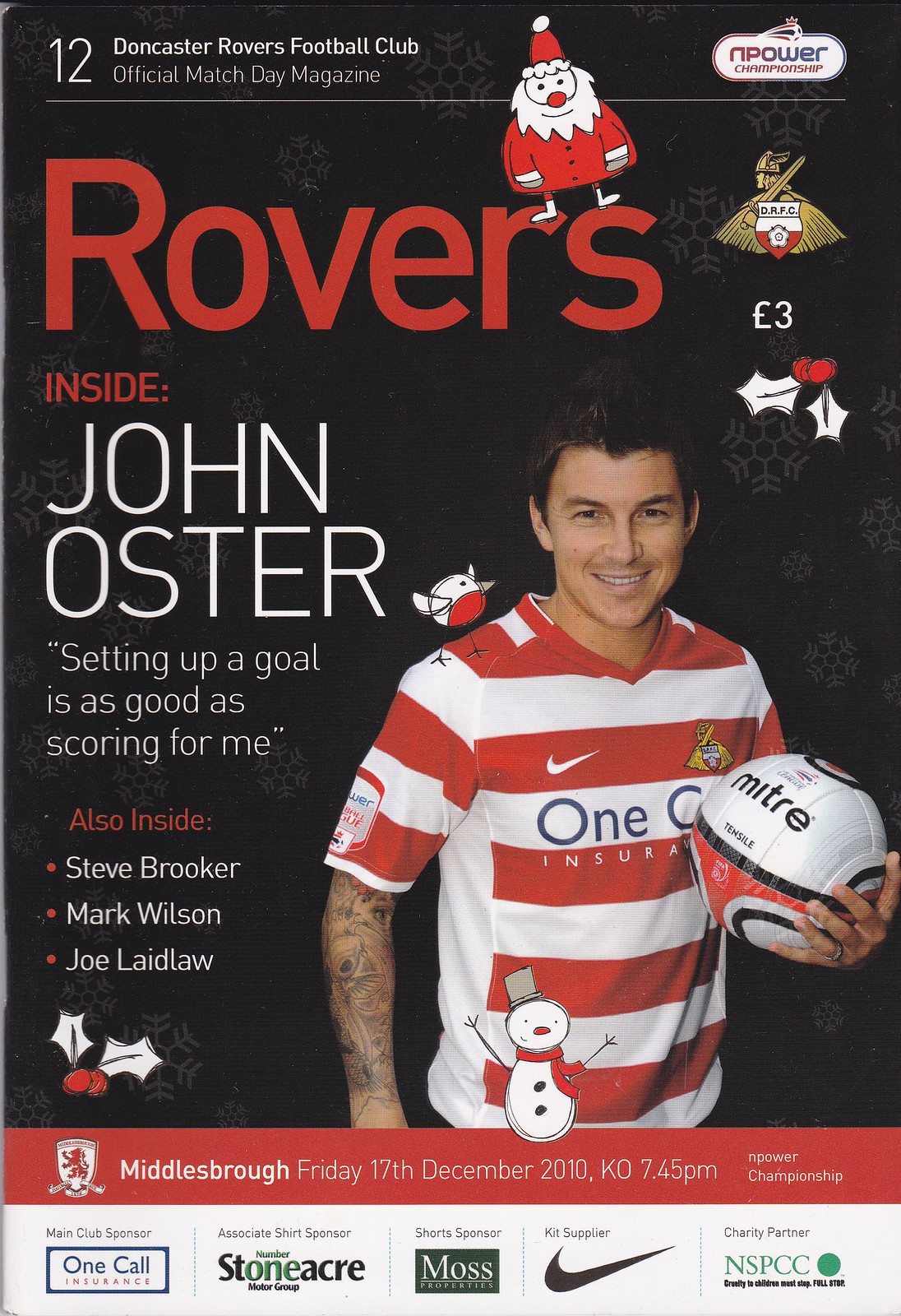This is a vertically aligned, scanned cover of the Doncaster Rovers Football Club Official Match Day Magazine, issue number 12. The background is black, and prominently displayed in the middle-right is a photograph of a soccer player. He has short dark brown hair, a toothy smile, and a tattooed right forearm hanging by his side. He is wearing a red and white striped jersey featuring a white Nike logo and blue text that partially reads "C". The player is holding a red, black, and white Mitre soccer ball against his chest with his left hand. Above his left shoulder is a cartoon image of Santa Claus with a red clown nose. To the left of the player, large red text reads "ROVERS," and below it in red letters is the word "INSIDE," followed by a larger white text that names the player, "John Oster." Beneath his name, a quote reads: "Setting up a goal is as good as scoring for me." The bottom section of the cover lists "Steve Brooker, Mark Wilson, Joe Laidlaw" in white text with red bullet points. Additionally, there is a smaller image on the bottom of a snowman with a grey top hat. The magazine details the match against Middlesbrough on Friday, 17th December 2010, with a kick-off at 7:45 PM, in the End Power Championships.